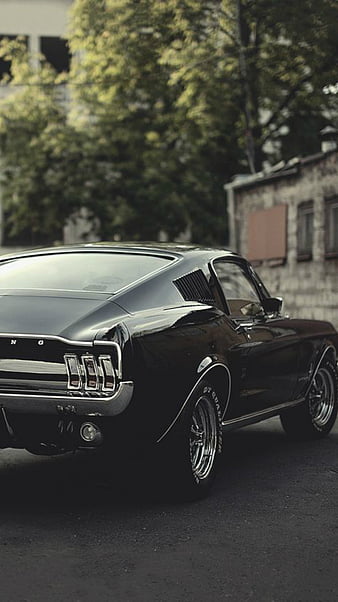The image features a meticulously polished black classic muscle car, likely a Ford Mustang, identifiable by the partial chrome letters "NG" on the rear. The glossy vehicle, a two-door model, boasts thin chrome trim around its wheel wells and vertical rectangular taillights. It’s parked on black asphalt near a dilapidated building with weathered shake-style siding, a boarded-up window, and possibly worn brick or cardboard-covered windows. The car's rear window is angled, and there’s a small round light below the rear bumper. The background includes blurry trees and the faint outline of another building, creating a contrast that accentuates the car's pristine condition amidst a neglected setting.